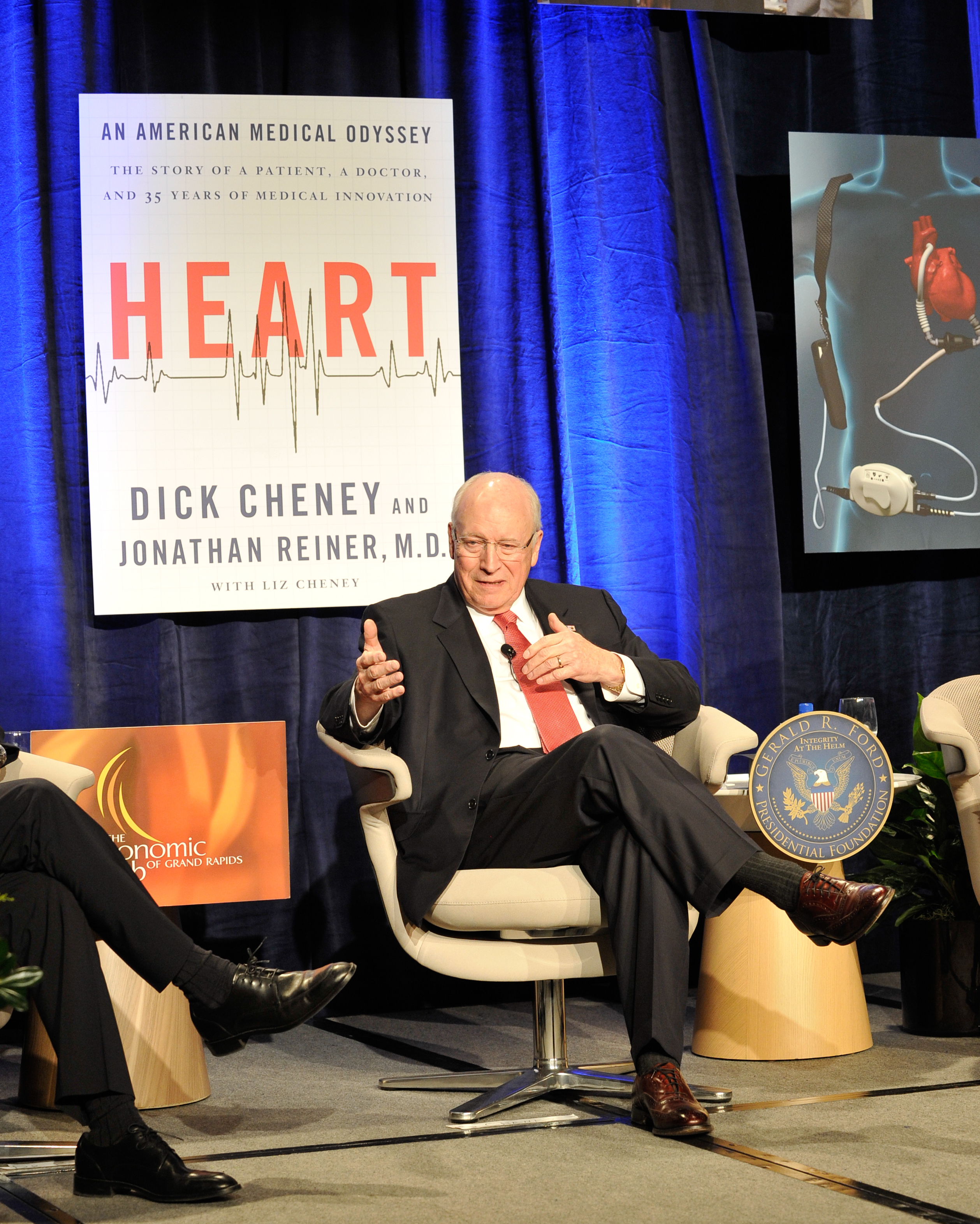The photograph captures Dick Cheney seated on a beige-colored swivel chair on a stage, engaged in what appears to be a discussion or Q&A session. He is dressed in a suit with a microphone clipped to his tie. The backdrop of the stage features a dark blue curtain with two prominently displayed poster boards. The right poster illustrates the outline of a person hooked up to various medical devices at the heart, waist, and shoulder. The left poster showcases the cover of a book titled "Heart: An American Medical Odyssey," co-authored by Dick Cheney, Jonathan Reiner, M.D., and Liz Cheney. This book details the narrative of a patient and doctor over 35 years of medical interventions. The photograph also includes multiple other individuals seated in armchairs, though only parts of them are visible. The setting suggests that Cheney is speaking at an event related to his book, likely discussing his personal medical experiences and the collaborative work with his co-authors.